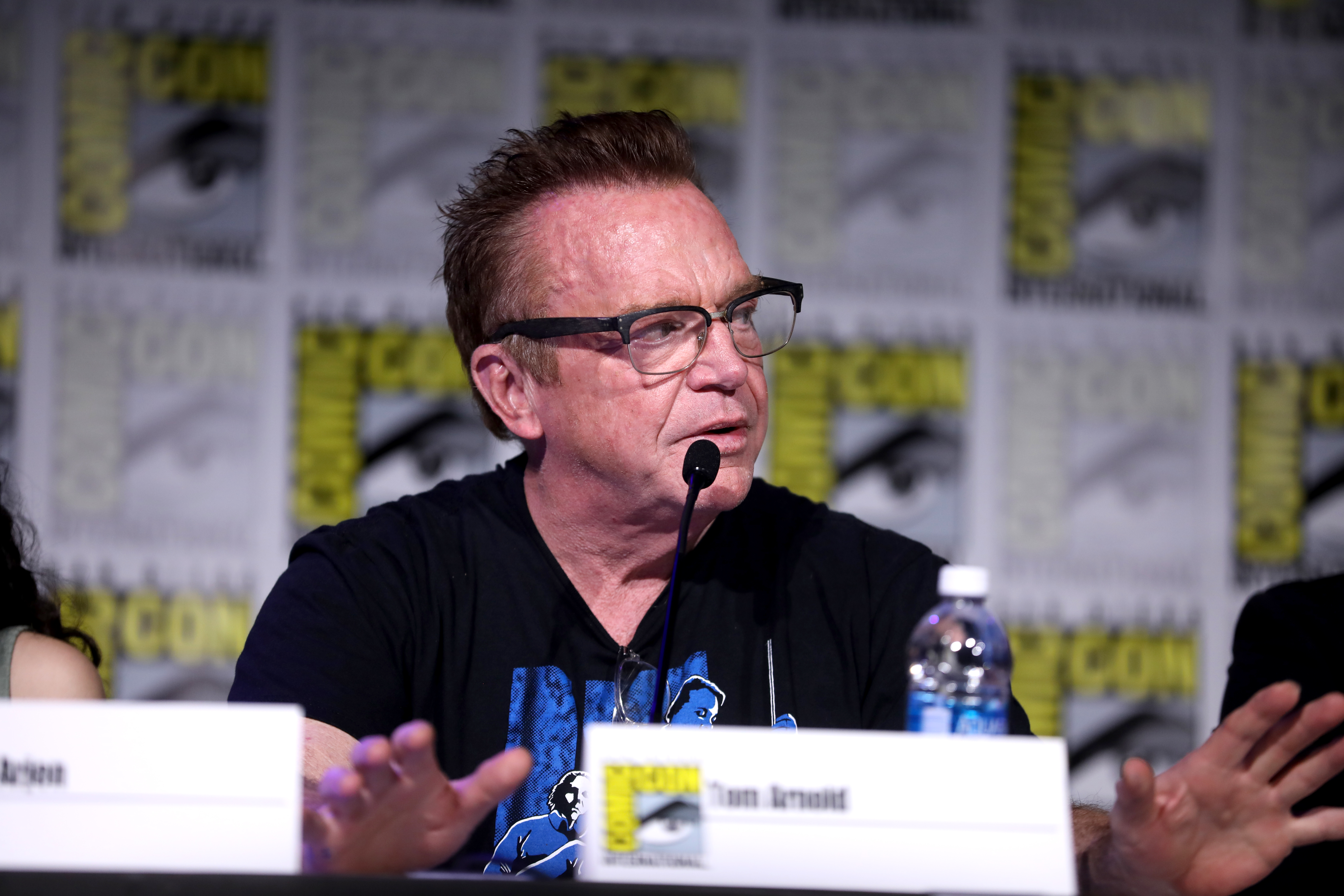In this detailed image, an older man with a full head of short brown hair, distinct wrinkles, and black aviator-style glasses with black frames is seated at a table, centrally positioned within the photograph. The photograph captures him from his lower chest to the top of his head. He is wearing a black graphic t-shirt featuring a blue design, partially obscured by a name card positioned in front of him. Additionally, a second pair of glasses hangs from his collar. His arms rest on the table with his wrists touching the surface while his hands are slightly raised, palms facing forward. 

In front of him, there is a clear plastic water bottle with a white cap and blue label. The text on the small white folded name card in the foreground is out of focus and illegible, and there is another similarly blurry name card visible to the left. Behind him, the background is dominated by a large poster or signage that reads "Comic Con," suggesting the setting is an indoor conference, possibly a panel discussion, with discernible colors including black, white, yellow, gray, tan, and blue.